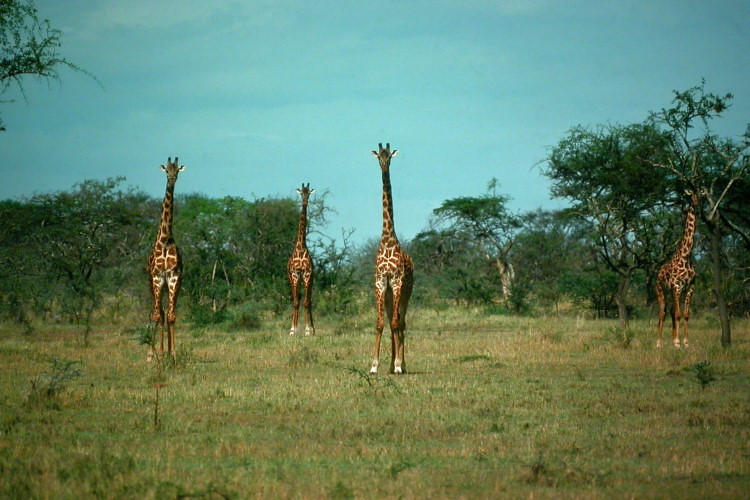In this photograph, a quartet of adult giraffes stands majestically on a grassy plain, facing the camera with an almost intentional poise. Their tall, slender necks adorned with the classic giraffe pattern of brown splotches on a white background extend upward prominently. Each giraffe is equipped with noticeable knobs or horns atop their heads and ears that splay outward. 

The setting is an outdoor, safari-like landscape, possibly somewhere in Africa. The ground is covered with a mix of light and dark green grass, dotted with occasional shrubs. A series of tall, deciduous trees with green leaves line the background, creating a somewhat continuous margin behind the giraffes. One of the giraffes is positioned closely enough to a tree that it reaches the high branches, nibbling on the leaves.

The sky overhead is a clear, light blue with a few wispy clouds. The overall scene suggests a serene and natural habitat with no signs of captivity. The giraffes, forming an evenly spaced ensemble, exhibit a calm demeanor as they gaze directly towards the camera, creating an impression of mutual curiosity and silent communication with the observer.